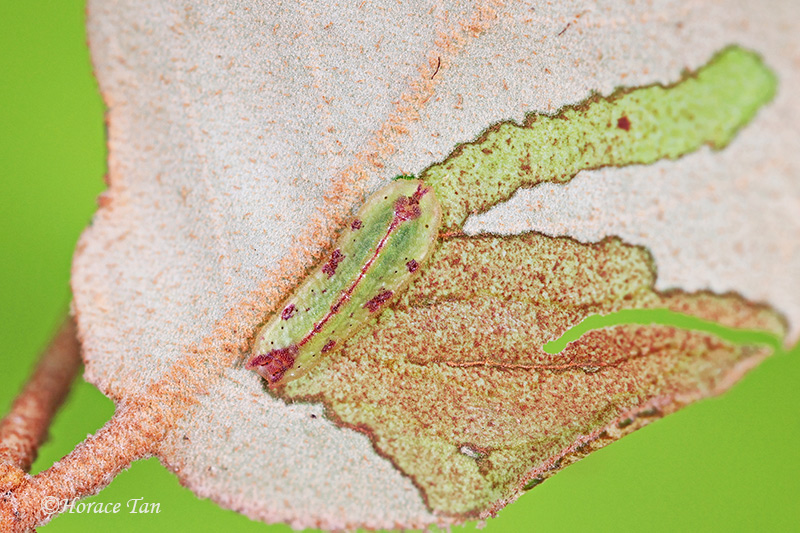This highly detailed, horizontal macro photograph by Horace Tan showcases the intricate textures and colors of a leaf. Dominating the right side of the frame, the leaf is tan with an intricate network of orangish-brown veins and a decaying stem. A significant portion of the leaf's surface is adorned with irregularly shaped patterns that resemble geographical states, primarily displayed in shades of tan, reddish hues, and yellow-greens. These patterns transition into a column of greens, highlighted by red and brownish mottling, stretching from the left-hand corner toward the center of the leaf. The entire image is set against a solid, out-of-focus chartreuse green background, which intensifies the leaf's complex visual texture. The photograph's emphasis on textures renders some areas velvety, others matte, and some scratchy with multicolored details. Notably, at the base of the leaf, an insect—potentially a cicada—is perched, exhibiting dark pink streaks, purplish splotches, and a texture that blends with the leaf's rich pointillism of browns, pinks, and greens. This intricate artwork leaves one pondering whether the astonishing details are the work of nature or an artist’s creative touch.